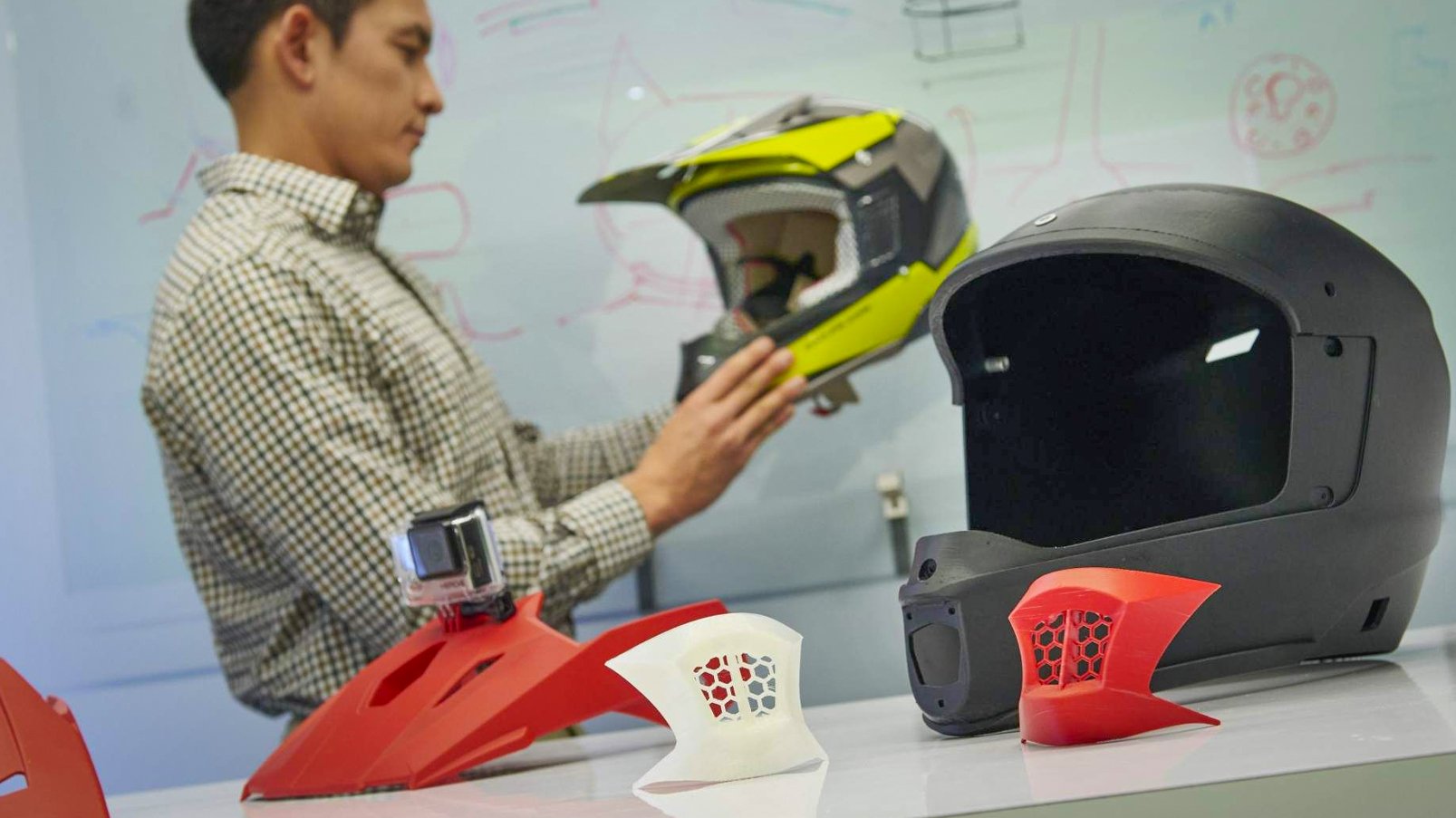In this photograph, a man in his 30s, wearing a brown plaid button-up shirt, is working on motorcycle helmet designs. He is holding a completed motorcycle helmet that is gray with yellow racing stripes and has a white inner padding. In the foreground, a white table displays various helmet components, including a sleek, modern-looking gray helmet shell with a yellow visor, a couple of face masks, and several red and white plastic pieces. Behind the man is a whiteboard adorned with various component sketches and designs, drawn in black and red, offering a glimpse into the meticulous design process.